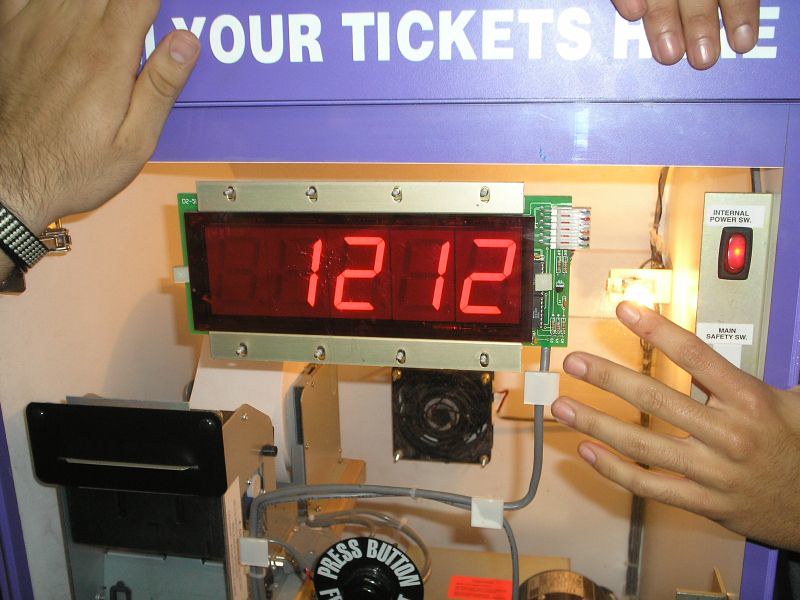The photograph features the inner workings of a ticket machine with its casing removed, revealing various electronic components. At the top of the machine, a purple background prominently displays the text "YOUR TICKETS HERE" in white, all-capital letters. The center of the machine exhibits an LED clock showing the time as 12:12 in red digits. 

Visible within the open case are intricate circuit boards, a computer fan, multiple cables, and an internal power switch. There is also a notable black button with the label "PUSH BUTTON" in white letters and a large red button on the upper right-hand corner. The machine appears to have components typically found in a parking meter, including a mechanism that might dispense tickets.

Three different hands are interacting with the machine: one on the upper left, sporting a black and gray wristband; another on the upper right, partially covering the word "HERE" with its fingers; and a third hand on the lower right, touching the glass or plexiglass section of the machine. This setup suggests a science fair or demonstration where viewers can explore the machine's inner mechanics.